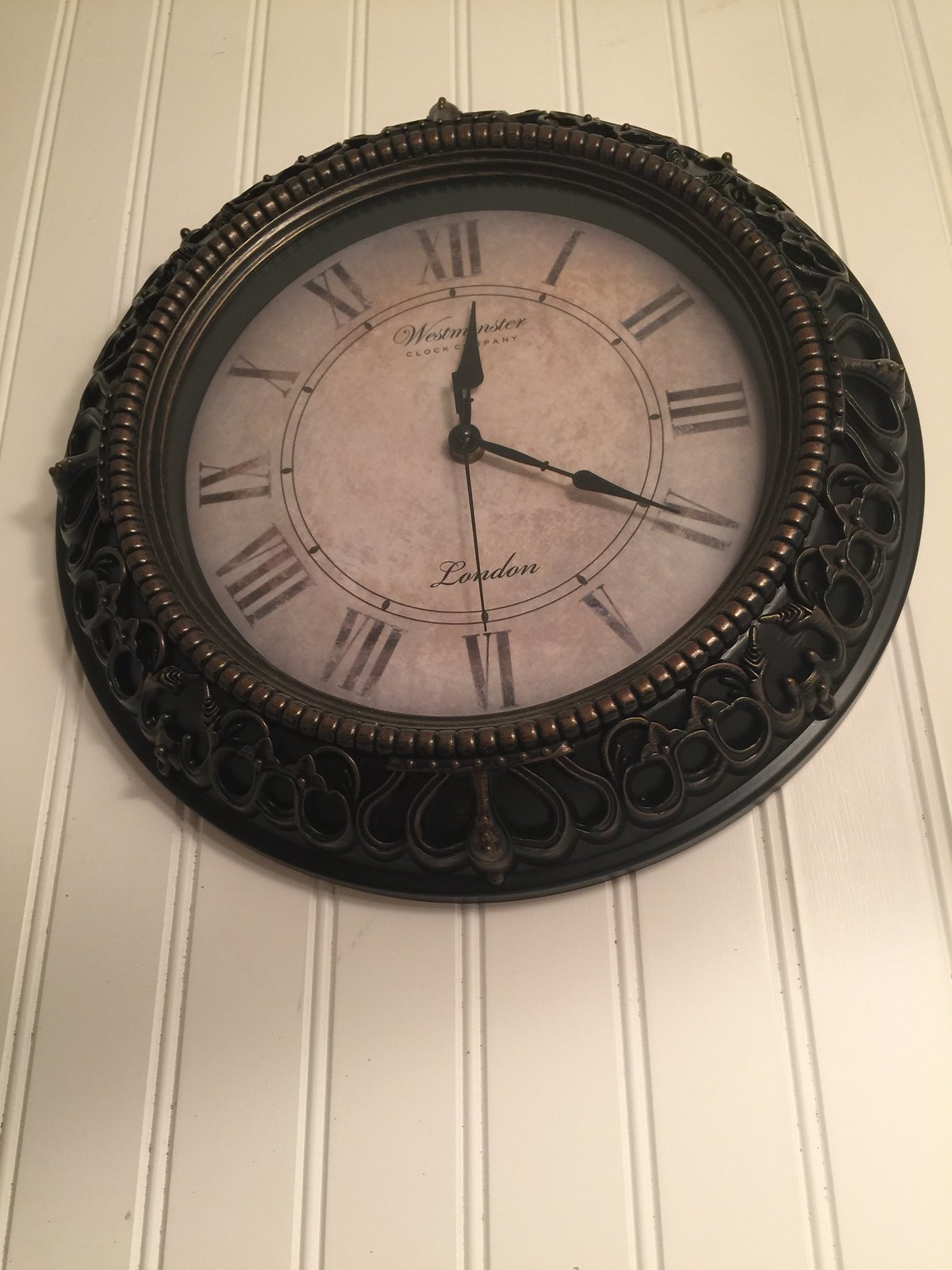This detailed photograph captures an antique wall clock hanging on a vertically paneled wooden wall, painted in an off-white to light beige color. The photograph is taken from a slightly lower angle, offering a close-up view of the clock. The clock's frame is an intricate, ornate dark metal with decorative accents, including curly Q designs and some lighter, bead-like elements closer to the clock face. The edge of the frame appears to be about three to four inches thick, exhibiting a textured look with hints of gold tones woven through the black metal.

The clock face itself has a distressed, dusty white appearance, adding to its antique charm. Roman numerals, once black but now somewhat faded, mark the hours. The top of the clock face features the text "Westminster Clock Company," while the word "London" is inscribed in cursive at the bottom. The clock's three black hands are particularly sharp and pointed; the hour hand points at 12, the minute hand at 4, and the second hand at 6, indicating the time is 12:20.